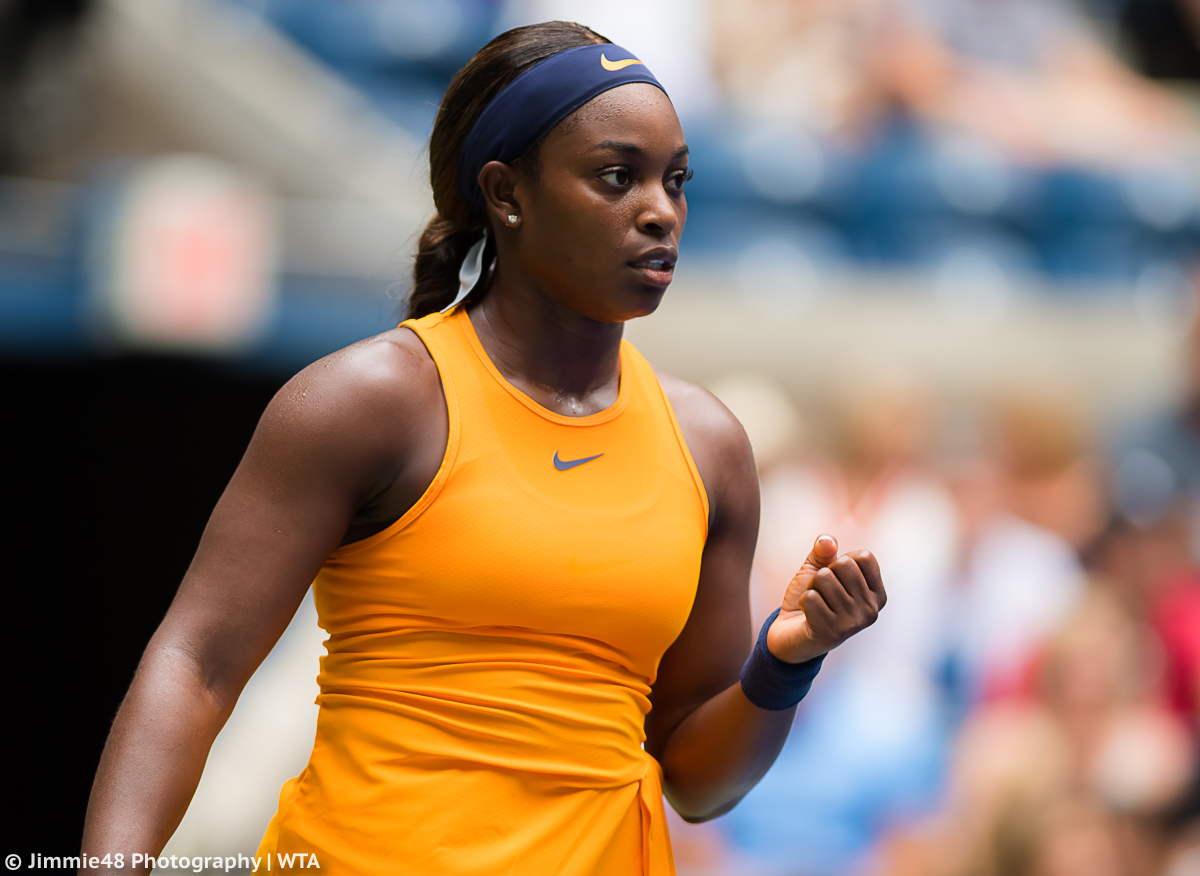The photograph features a focused African-American female athlete, likely a tennis player, centered against a blurred background that hints at a crowd of spectators. She's wearing a yellow, sleeveless Nike tank top with a blue swoosh right below the neckline, paired with a dark blue headband that also sports a yellow Nike swoosh. Her hair is pulled back into a twisted ponytail, secured with a white ribbon, and she has a small earring in her right ear. The player strikes a triumphant pose with her left hand fisted and elbow bent, displaying a serious yet slightly smiling expression. The overall scene is outdoors on a tennis court. At the bottom left corner of the image, there is a copyright notice that reads, "Jimmy 48 Photography WTA." The colors prominent in the image include black, brown, white, orange, gray, dark blue, red, pink, and tan.